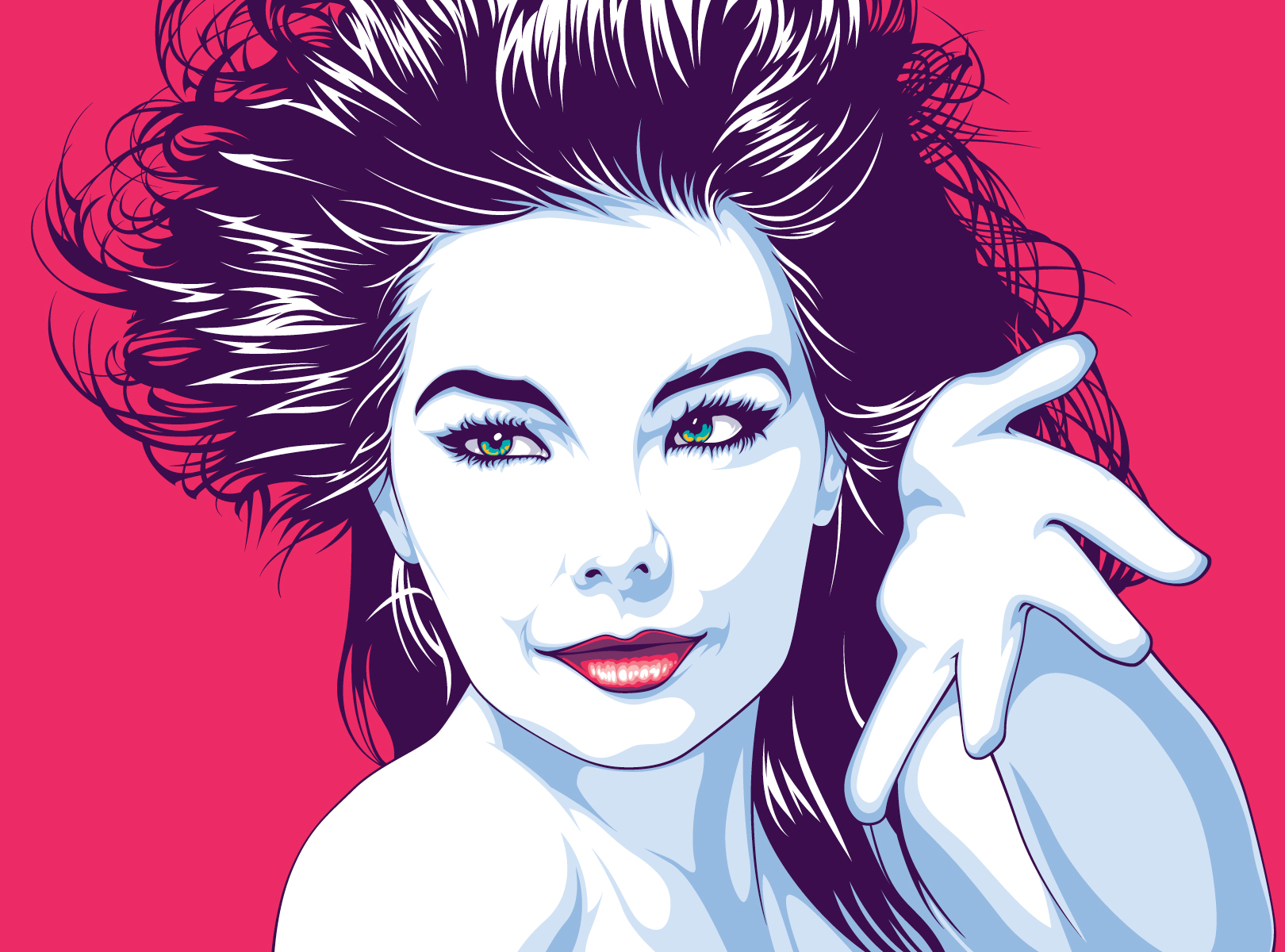This image is a cartoon drawing of an artistic rendition of a glamorous woman set against a solid red background. The woman, who exudes a striking and exotic beauty, has very pale, almost porcelain white skin that appears shiny. Her facial features are accentuated with bold, dark red lipstick and striking light green, almost emerald eyes framed by very sharp, curved eyebrows and dark eyeliner. Her wild, teased hair, reminiscent of a Pat Benatar rock star look, is primarily black with shiny white streaks that add to its dynamic appearance. The woman is depicted from the shoulders up, with her bare shoulders suggesting she is not wearing any clothes or jewelry. Her left hand is partly raised and extended, as if reaching toward someone, while her gaze is directed upwards to the left, adding an element of intrigue and elegance to her pose.